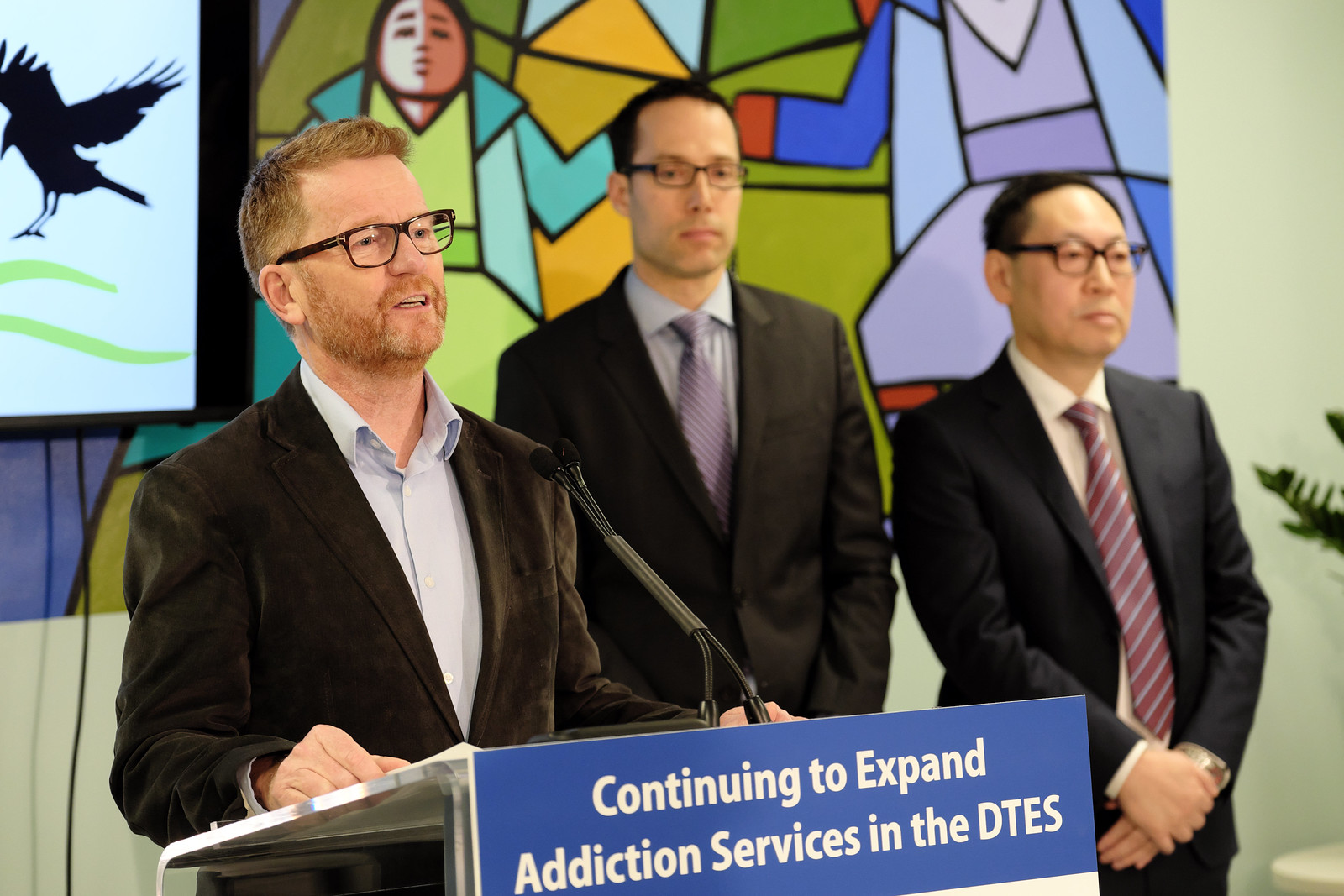This rectangular indoor photograph features three men, all wearing black glasses and standing in front of a wall decorated with what appears to be either a mural or stained glass artwork. Central to the image is a man of Caucasian descent, positioned at a podium with microphones angled toward his face. He sports reddish-brown facial hair and is attired in a brown suede jacket over a light blue button-up shirt, notably without a tie. The podium, metal and tilted slightly upward from left to right, exhibits a blue sign with white text reading "Continuing to Expand Addiction Services in the DTES."

To his left (our right), are two men of Asian descent, both clad in suits and ties. The man on the left appears taller and stands attentively observing the speaker, while the one next to him gazes out into the audience with his hands clasped in front of him, listening intently. The background incorporates a complex array of imagery, including a semi-visible depiction of a taller person and child, and an element that resembles a black raven situated on the far left, possibly part of a TV screen.